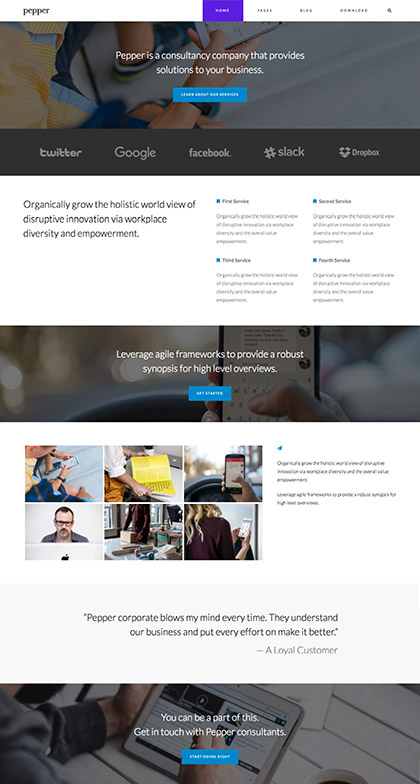This image is a screenshot most likely taken from an iPad, as suggested by its dimensions. The screenshot is from the website of a company named Pepper. At the top of the image, the company's name is displayed in a stylized font. Due to the small and somewhat blurred text, readability is a challenge. However, it is clear that a menu is present at the top, with one of the items highlighted in purple.

The main section of the image features a photograph of an individual sitting down and holding a mobile phone, though only their lower half and feet are visible. Superimposed over this image is text stating, "Pepper is a consultancy company that provides solutions to your business," written in white. Below this, a blue button is displayed, although the text on it is not legible.

Further down, the website showcases logos of prominent businesses including Twitter, Google, Facebook, Slack, and Dropbox. Underneath these logos, on a white background with black text, it reads, "Organically grow the holistic worldview of disruptive innovation via workplace diversity and empowerment." The bottom section of the screenshot displays additional images of people, suggesting a focus on community or team dynamics.